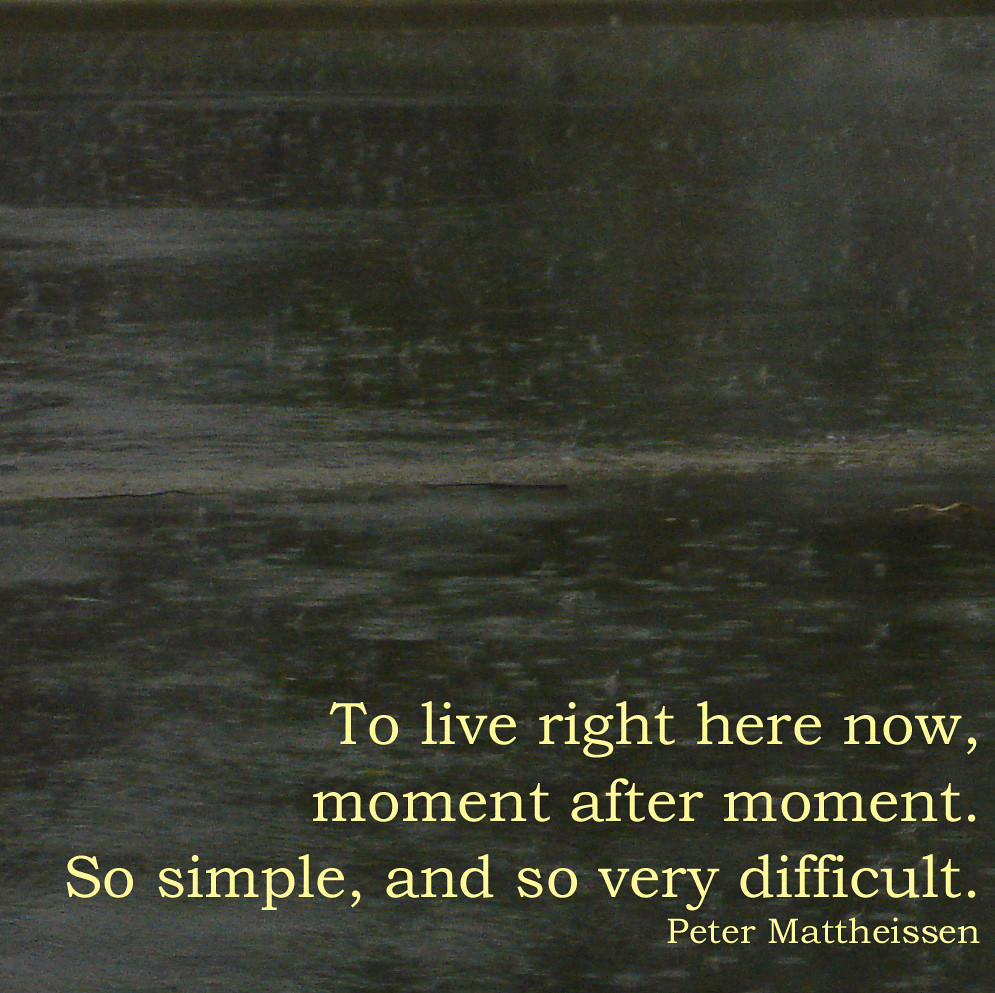The image is an inspirational poster set against a dark, rainy backdrop, capturing a muted, blurry scene of a flooded ground or body of water. The background features a mix of dark gray, brownish, and greenish tones, creating a somber, reflective atmosphere. Prominent yellow serif text, likely in a font resembling Times New Roman, is positioned towards the bottom right of the image. The text reads: "To live right here now, moment after moment, so simple and so very difficult." Beneath this quote, in slightly smaller yellow font, is the attribution: "Peter Matthiessen." The overall image, while having a dark and grainy appearance, conveys a high clarity of purpose and drives a contemplative mood through its composition and message.